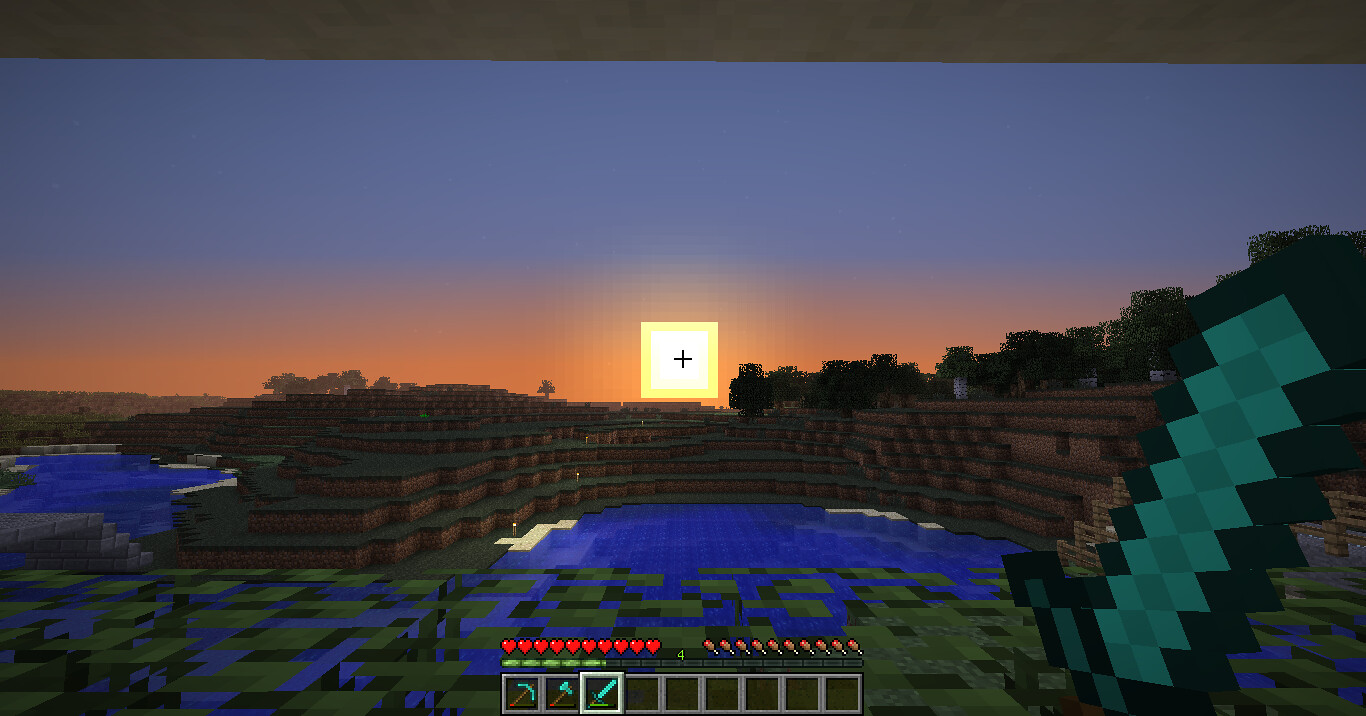This digital artwork captures a scene reminiscent of a computer game or virtual landscape. The central focus is a terraced green hillside, bathed in the warm glow of either sunrise or sunset. A gradient sky transitions smoothly from deep blue at the top to vibrant oranges and yellows near the horizon, enhancing the serene atmosphere. Prominently positioned in the center of the image is a bright yellow square, intersected by a black cross, seemingly anomalous atop the rolling hills.

The hillside itself is a lush tapestry of greens, browns, and specks of gold, leading the eye downward to a peculiar arrangement of blue squares and rectangles along the bottom, which likely represent a body of water. To the right, a staircase-like formation of green diamonds descends diagonally from top to bottom, each diamond composed of two shades of green, totaling about ten stacked cubes. This intricate arrangement adds a layer of geometric complexity to the scene, inviting closer inspection.